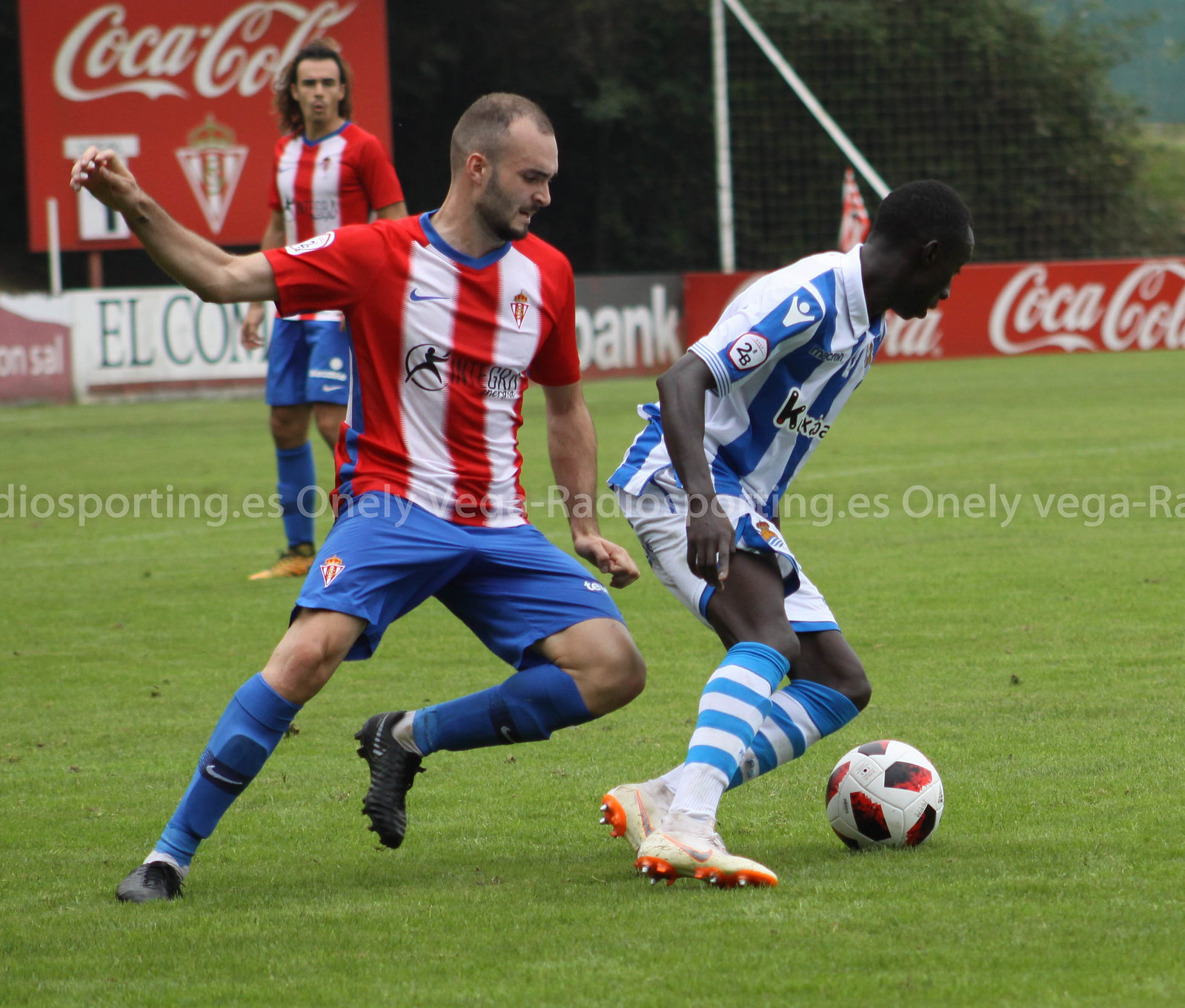In this professional photograph taken on an overcast day, three soccer players are captured in action on a vivid green grass field. Two players, one a Caucasian man and the other obscured but also wearing a red and white jersey with blue shorts and blue socks, are about to kick a white football adorned with black and red designs. A third player, an African-American man dressed in a blue and white jersey with matching striped socks, is moving toward the ball. Behind them, a boundary wall with advertisements featuring brands like Coca-Cola and E-L-Com is visible, along with a metallic fence and lush green trees. A watermark reading "vega-radio-sporting.es" spans the center of the image, marking it as an official snapshot.